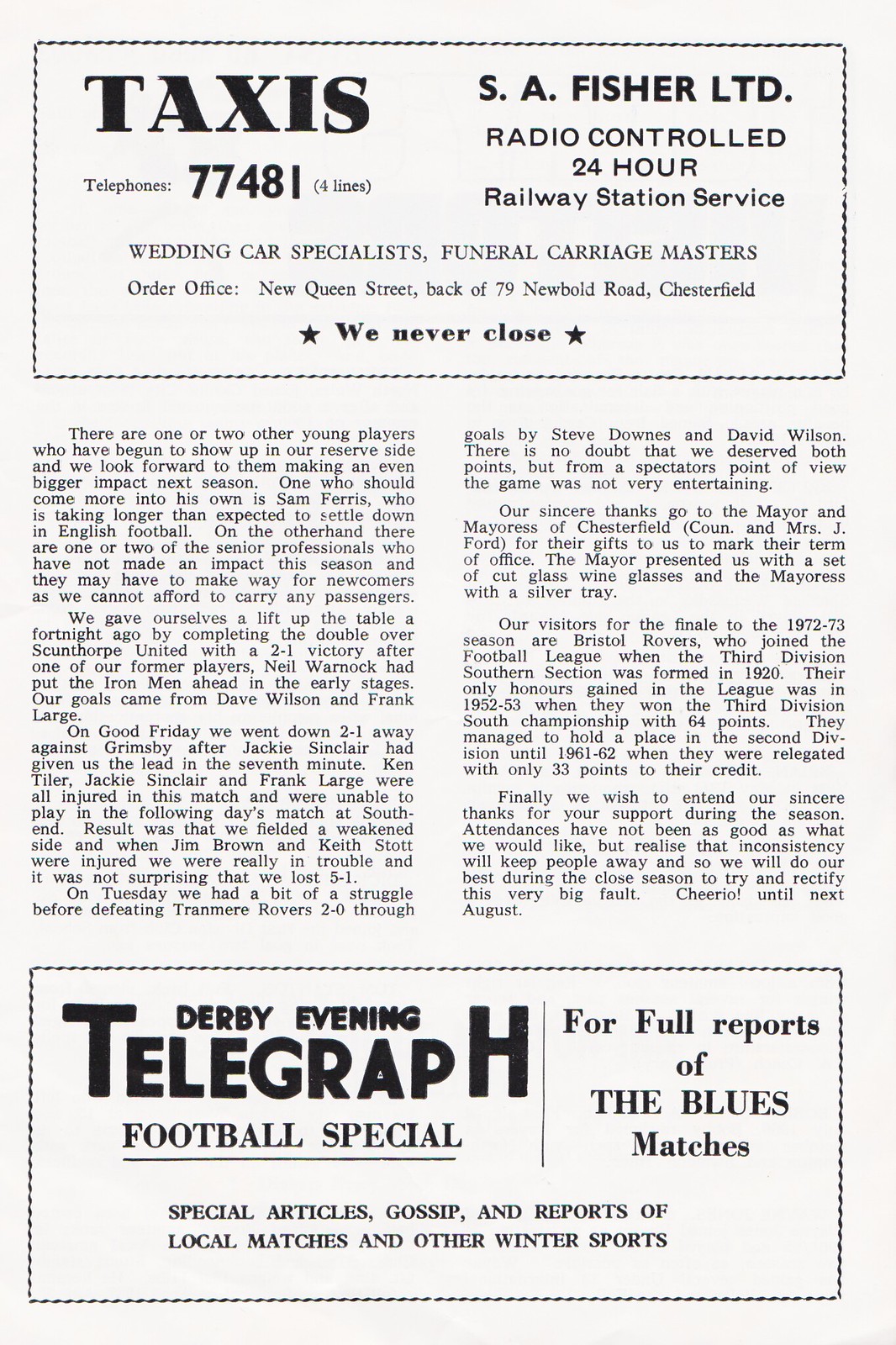This tall, rectangular photograph showcases a page from a newspaper or magazine, with a light gray, off-white background. At the top, there is a swirly, horizontal rectangle outlined in black, containing the bold, all-caps text "TAXIS." To the right within this box, it reads: "S.A. Fisher LTD Radio Controlled 24-Hour Railway Station Service." Just below, additional text details, "Wedding Car Specialist Funeral Carriage Masters," followed by, "Order Office, New Queen Street, back of 79 Newbold Road, Chesterfield." The section concludes with the bold phrase "WE NEVER CLOSE," flanked by two black stars. 

Beneath this advertisement, the central area of the image contains two columns of text from an article, too small to discern specific words. 

At the bottom of the image, there is another outlined, rectangular section with bold text in the top left corner reading, "Derby Evening Telegraph Football Special." A line under this title splits the box, with content on the right side stating: "For full reports of the Blues matches." Beneath this, spanning the width of the box, it continues: "Special articles, gossip, and reports of local matches and other winter sports." This section appears to be an advertisement or informational segment related to football match coverage.